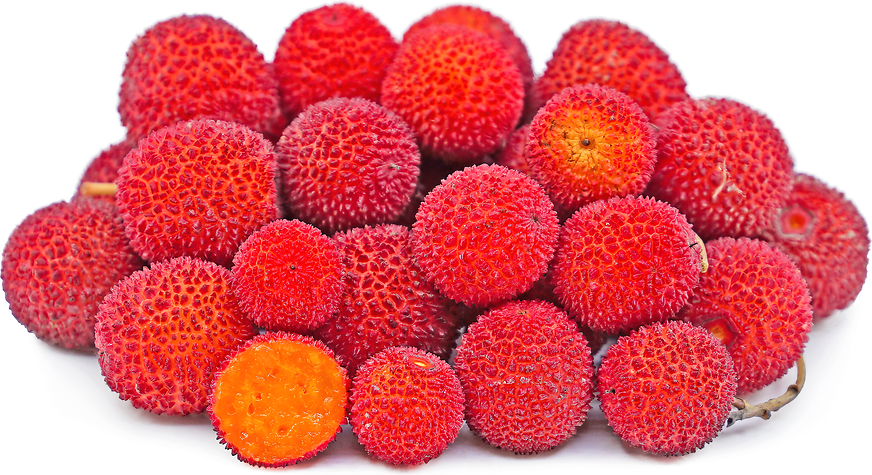In this image, we observe a prominent mound of a unique, unfamiliar fruit, occupying almost the entirety of the frame against a pristine white background. The central pile, composed of multiple layered fruits stacked nearly four high, draws immediate attention. Each piece of fruit showcases a spiky, sandpaper-like texture, with a striking bright red color that darkens to a deep red at the tips of the spikes. The fruit's base exhibits shades of orange and yellow. 

Towards the bottom left of the arrangement, one fruit is cut open, revealing a vivid orange, peach-like flesh inside. This cross-section gives insight into the fruit’s texture, which bears a resemblance to that of a grape or peach, enhancing the overall visual appeal. Additionally, a stem can be noted in the bottom right corner of the pile, suggesting the fruits are still somewhat attached. The clear, detailed composition of the image makes it ideal material for a food blog or could even be seen on a supermarket shelf display, underscoring both its aesthetic and informative qualities.